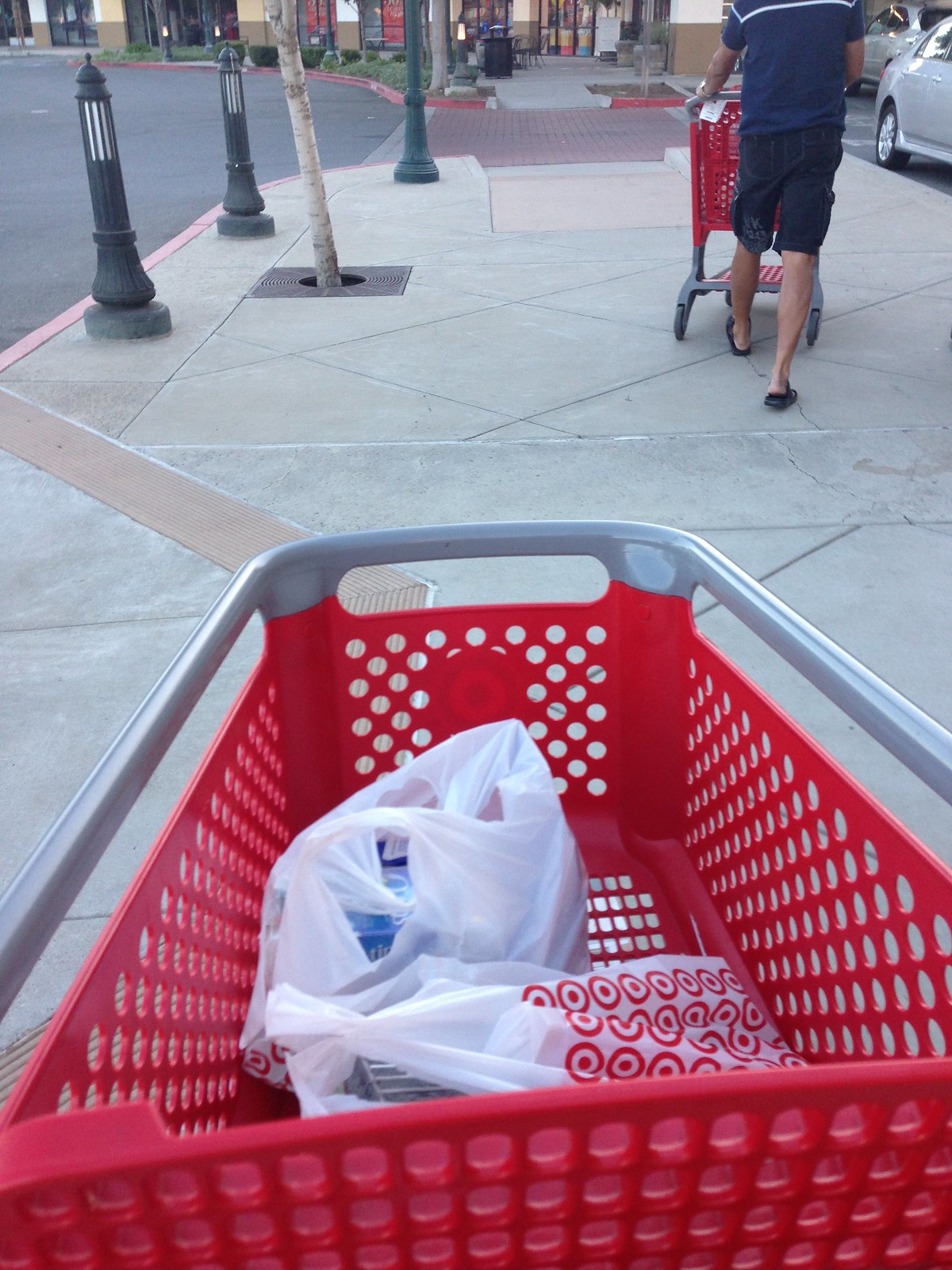This vertical, color photograph captures a Target shopping cart being pushed along a sidewalk from the point of view of the person pushing it. The red shopping cart, with its characteristic circular holes and a gray metal railing on top, contains two white plastic bags adorned with the Target bullseye logo. The contents of the bags are indiscernible. The grayish-tan concrete sidewalk features a red-brick crosswalk up ahead and a curb with a red edge. In the background, to our left, there are black metal streetlamps and a small tree emerging from a grating. Ahead on the path, a person clad in a blue short-sleeved shirt with a white stripe, blue jean shorts, and flip-flops is pushing a similar red cart. This person’s left arm is extended to grip the cart while their right arm is visible up to the elbow, with their steps captured in motion – left foot forward, right foot trailing. Partly visible cars, including a white one, are parked on the top right side near the storefronts, which have clear glass doors and green plants inside. The scene unfolds during the daytime, under subdued lighting, making the environment brightly lit but not glaring.